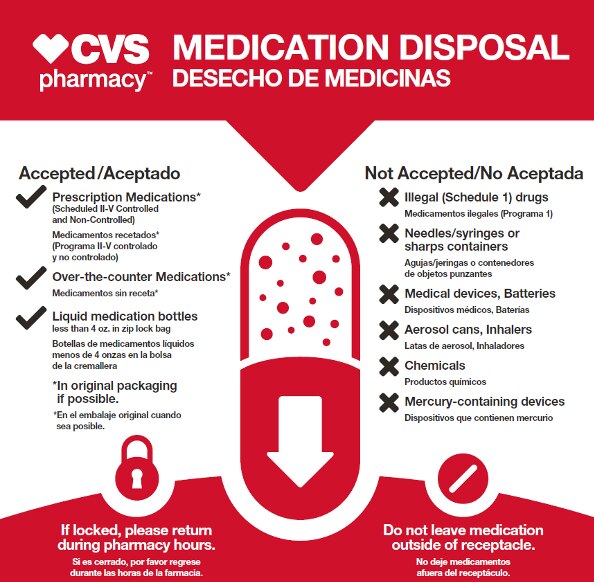This is a detailed poster from CVS Pharmacy about medication disposal. At the top, a red banner with a triangular bottom displays the CVS Pharmacy logo along with the text "Medication Disposal" and its Spanish translation. The center features a large capsule pill graphic with a clear top filled with dots, pointing downward like an arrow. 

To the left of this image, there is a list of accepted items which include prescription medications (Schedules II-V, both controlled and non-controlled), over-the-counter medications, and liquid medications in containers of less than four ounces, preferably in their original packaging and placed inside a Ziploc bag. Each accepted item is marked with a check.

To the right, the poster lists items that are not accepted, marked with an X. These include illegal Schedule I drugs, needles, syringes, sharps containers, medical devices, batteries, aerosol cans, inhalers, chemicals, and mercury-containing devices.

At the bottom of the poster, another red banner instructs, "If locked, please return during pharmacy hours." On the right side, additional instructions state, "Do not leave medication outside of receptacle." The font throughout the poster is black against a white background, ensuring clarity. This comprehensive guide aims to assist customers in disposing of their medication safely and correctly.